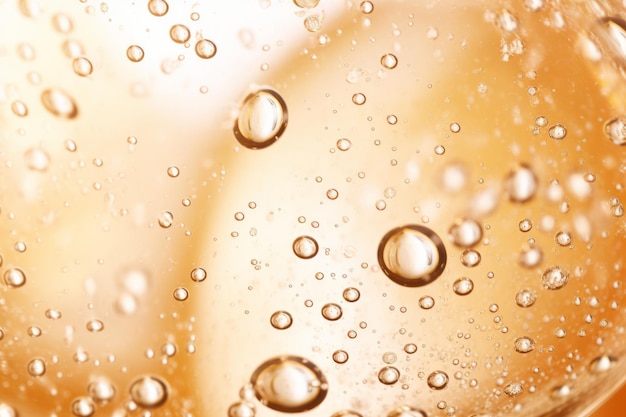The image is an extreme close-up photograph that captures a scene through a glass or clear surface covered in droplets of water. The background features a soft, golden brown color which is reflected in the water droplets, giving them a similar golden brown hue. The droplets vary in size, with some being large and outlined in dark brown, while others are smaller or even microscopic. In addition to the condensation, there are small white dots throughout the image that resemble bubbles. Behind the glass, the blurred yet discernible shape of human buttocks can be seen, suggesting the scene might be in a shower stall. The visible cheeks and crack suggest the body is somewhat curvy, likely indicating a female figure.